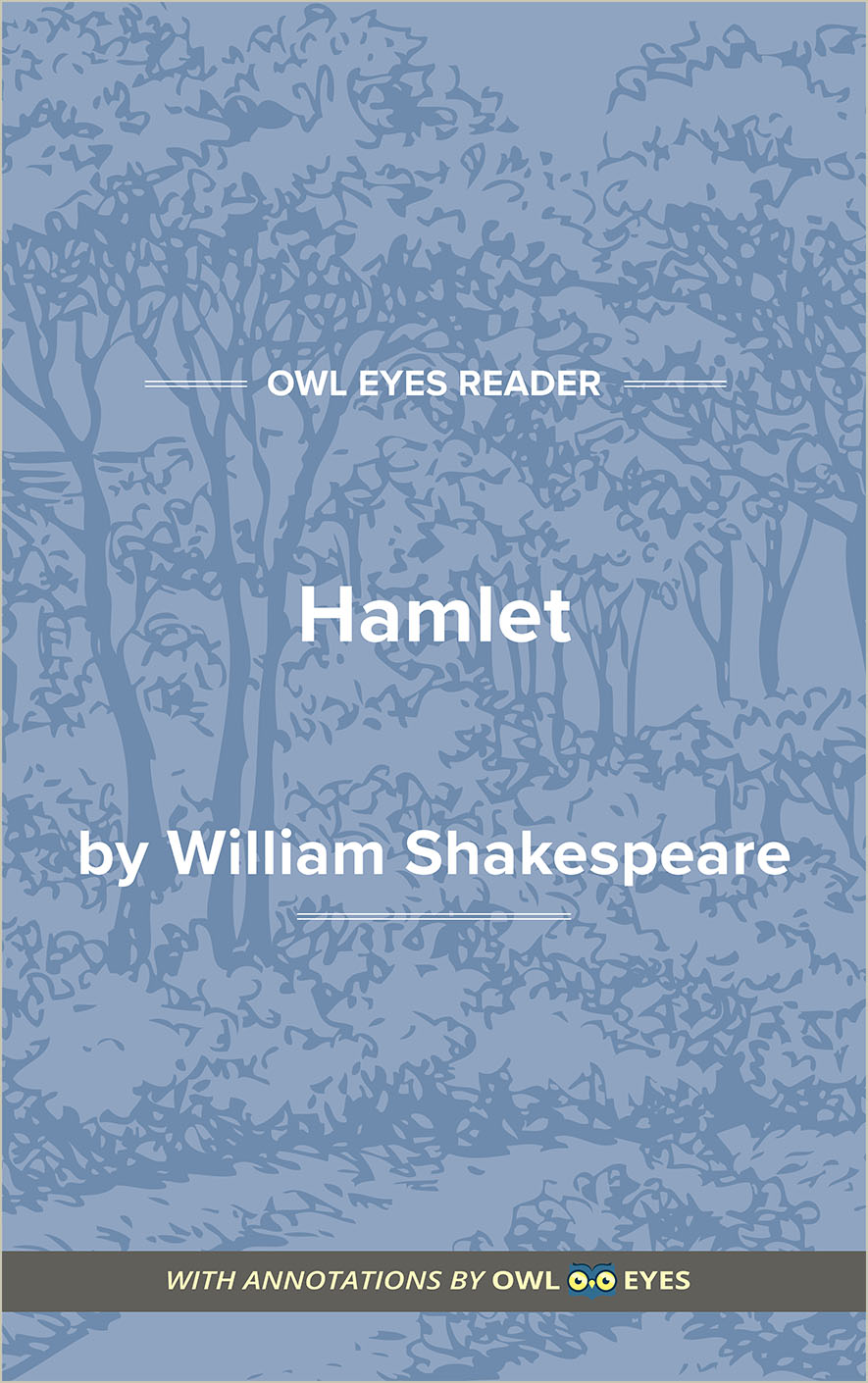This is a detailed description of the book cover. The cover features a soft pastel blue background with subtle, light grayish-blue line drawings depicting thin trees, shrubs, and a path winding from the bottom left corner. At the top of the cover, the text reads "Owl Eyes Reader," with a decorative dashed line framing this title. Centered in bold text is "Hamlet," with "by William Shakespeare" just below it. At the very bottom, a gray band states "with annotations by Owl Eyes," accompanied by small illustrations of owl eyes. The overall design is minimalist, featuring light blue hues and delicate illustrations creating a serene woodland scene.